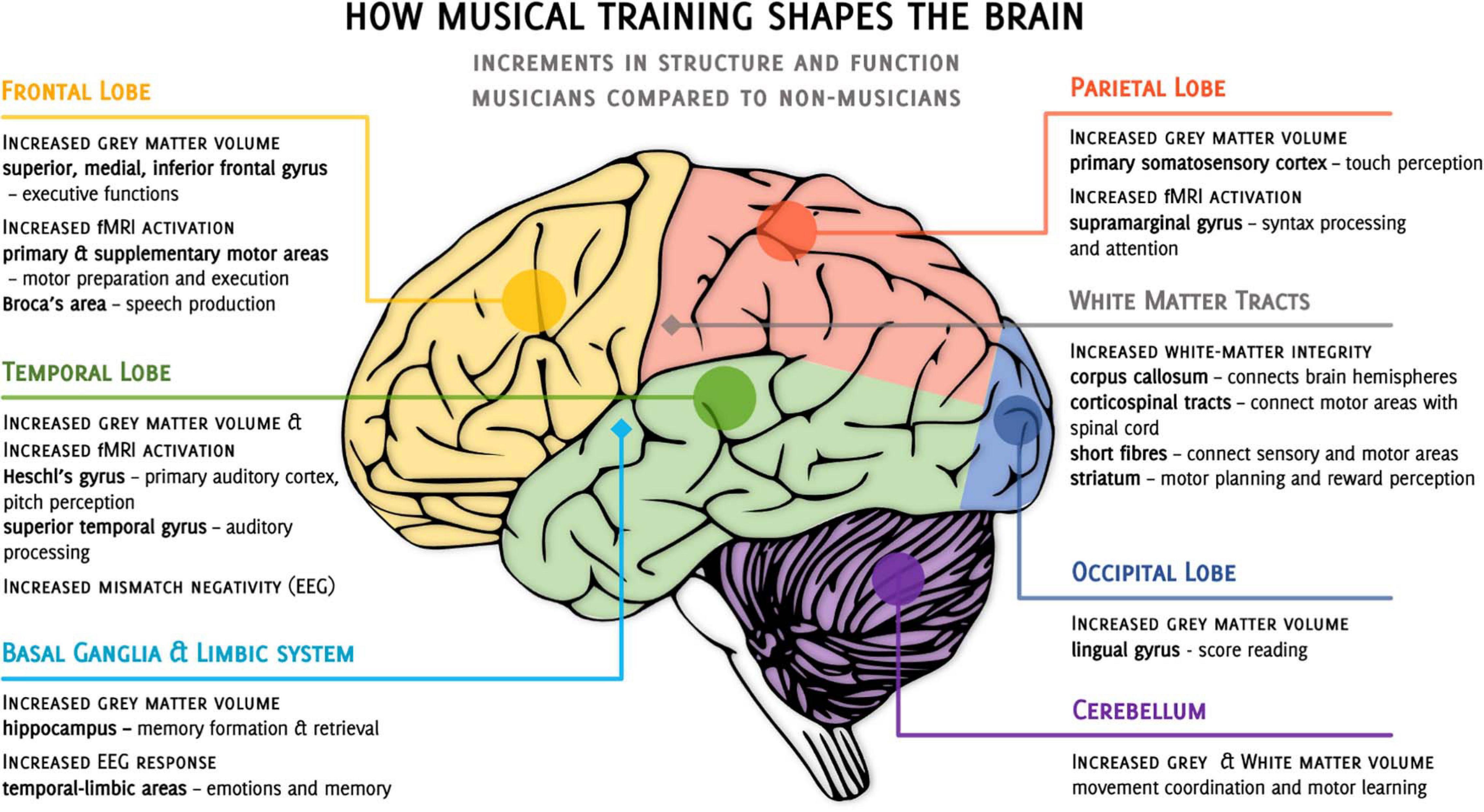This image is an informational graphic depicting how musical training affects brain structure and function, comparing musicians to non-musicians. Titled "How Musical Training Shapes the Brain," with a subtitle, "Increments in Structure and Function, Musicians Compared to Non-Musicians," the graphic features a color-coded diagram of the brain with various labeled regions. 

- The **frontal lobe** is highlighted in yellow.
- The **temporal lobe** is shown in olive green.
- The **basal ganglia and limbic system** are marked in teal.
- The **parietal lobe** is indicated in an orange or reddish hue.
- The **white matter tracts** are depicted in gray.
- The **occipital lobe** is shown in dusty blue.
- The **cerebellum** is colored in purple.

Each labeled region has a line pointing to its respective area on the brain diagram, illustrating how musical training leads to structural changes, primarily noting increases in gray matter volume in these regions.